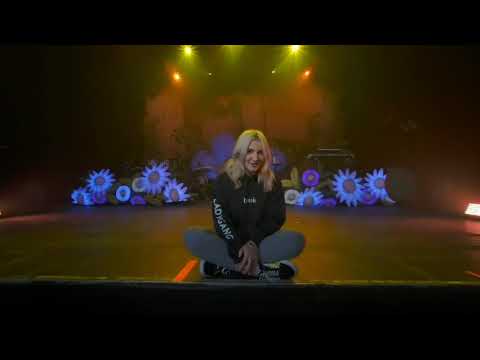In this image, a young woman, approximately 25 years old, sits cross-legged at the center of a stage, looking directly at the camera. Her hair is blonde, and she is dressed in a black hoodie with "Lady Gang" written on the sleeves in white letters, gray pants, and black and white sneakers. The stage is black with red lines, and in the background, a diverse array of artificial flowers in hues of blue, purple, yellow, and white are illuminated by various stage lights. The setting appears to be indoors at a performance center or concert venue, featuring a backdrop that includes bluish smoke and what looks like stage props representing buildings. The overall scene is framed by black borders at the top and bottom, adding to the dramatic ambiance of the photograph.